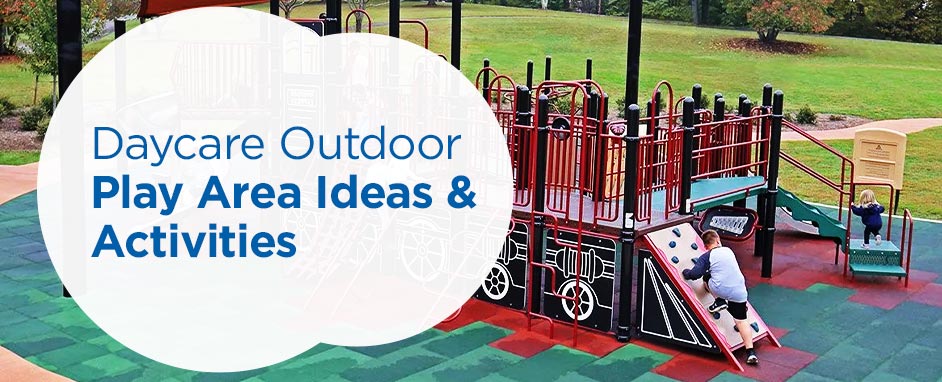This promotional image for daycare showcases an inviting outdoor play area designed for children. On the left, a white and blue logo prominently reads "daycare, outdoor play area ideas and activities," featuring a larger and a smaller bubble, contributing to the modern branding. The background reveals a lush, grassy park with leafy trees, presenting a serene environment.

The focal point is an extensive playground with a train locomotive design. The playground area includes green foam mats and red concrete walkways. Children are seen actively engaging in various activities: one child is climbing a ramp with holes, another navigates through stairs, and a young boy in a white T-shirt with blue sleeves and black shorts ascends a small rock wall. Nearby, a blonde-haired girl climbs the stairs.

The structure comprises green steps, red handrails, and black tubular posts with rounded tops for safety. The equipment is surrounded by a tan border, adding to its visual appeal. The overall vibrant colors and detailed textures highlighted in the play area - including the red metal handrails and safety bars - clearly depict the daycare's emphasis on providing a safe, fun, and engaging environment for children's outdoor activities.